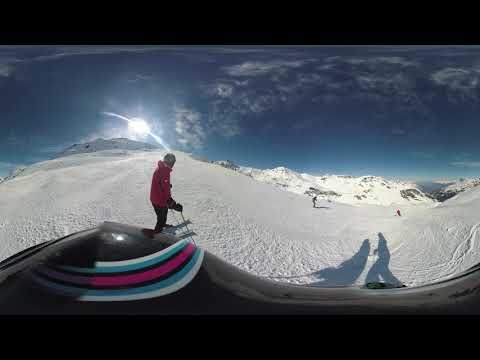A 360-degree panoramic image captures a skier in a vibrant red jacket with black pants, black gloves, and equipped with ski poles and skis, standing near the camera, possibly on a helmet or a selfie stick, at the top of a snowy slope. There's a shiny black object, likely part of the helmet or camera mount, visible at the bottom of the image. The skier might be sporting goggles and a hat or helmet. The panoramic view emphasizes the stark white snow under a deep blue sky with scattered wispy clouds and a bright sun peeking over snow-covered mountains in the distance. The perspective is slightly distorted, making objects closer to the camera appear larger, while those further away appear smaller. Shadows of at least one skier stretch across the snow, and further down the groomed slope, additional skiers can be seen, albeit less distinctly. The scenic backdrop provided by the sunlit mountains and clear blue sky highlights the elevated, serene location of this winter sports activity.